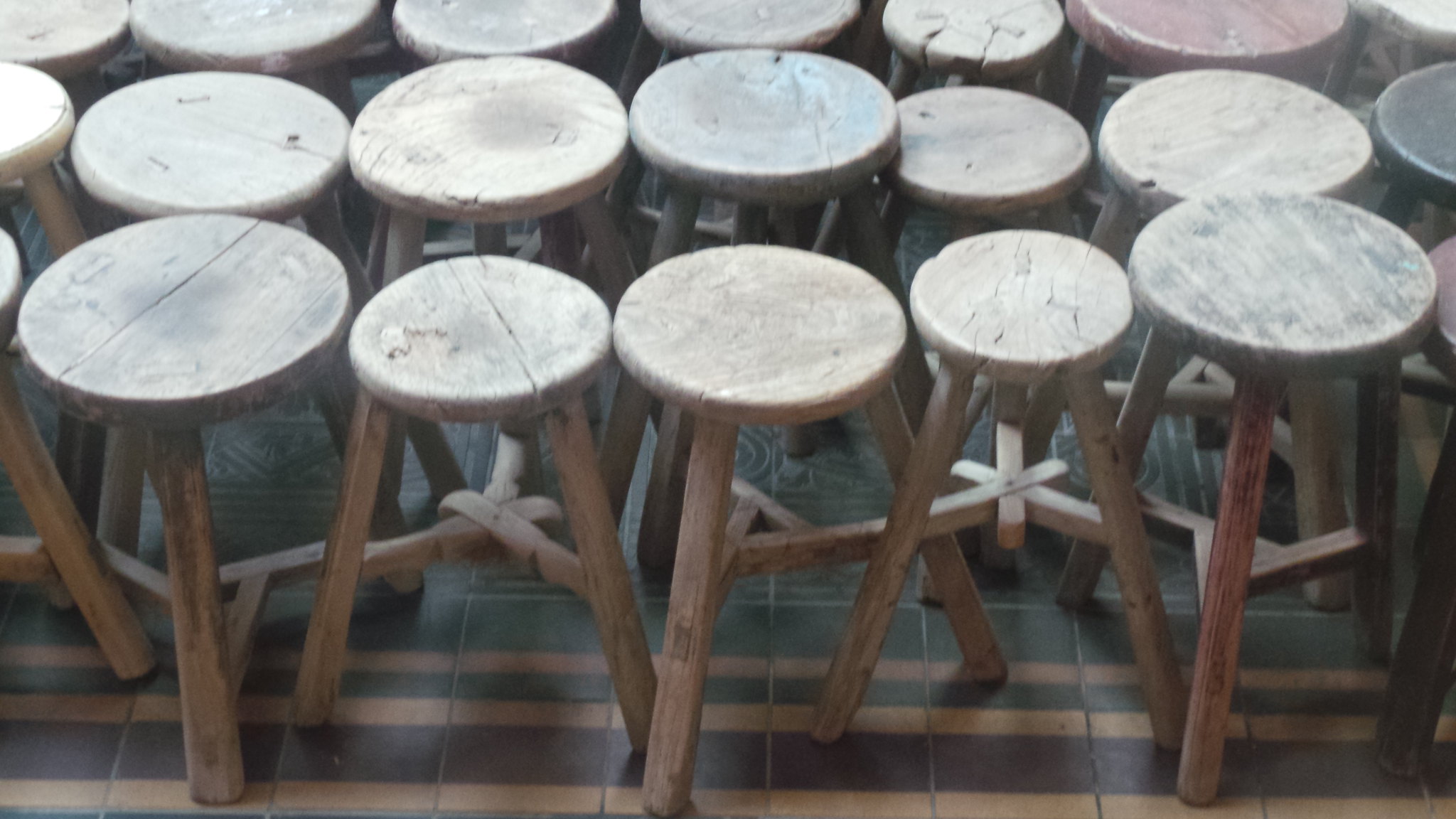This horizontal, rectangular photograph features a dense assembly of wooden, three-legged stools, packed closely together on a striped tile floor. The tiles are organized in parallel bands of dark red, beige, and black, running horizontally across the image. The stools are systematically arranged in rows; two complete rows with five visible stools each, and partially visible stools on either end suggest the rows extend beyond the image's borders. Additionally, there is a partial row at the top of the frame, with more stool legs peeking through the gaps, hinting at further rows beyond the photograph's top boundary. The stools, intended for use at a counter or high table, are uniform in their natural wood appearance, although a few show signs of wear with visible cracking on the round seats. Contrary to the initial impression of some stepstools, these are all seating stools, primarily wooden, mostly retaining their natural finish with a speculative few possibly appearing in darker hues or green due to lighting contrasts. The meticulously detailed composition captures the mass of stools while highlighting the characteristic striped design of the tile floor below.